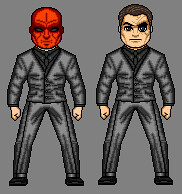This image is a detailed and stylized character drawing, featuring two versions of Arnold Schwarzenegger as the Terminator. Both characters are portrayed in gray suits with black shirts underneath, suggesting a coordinated or team-like appearance. The character on the left has a strikingly red face, reminiscent of the Red Skull, while the character on the right maintains a more typical facial appearance. The depiction, likely computer-generated or artistically drawn, emphasizes the iconic nature and legacy of Schwarzenegger's Terminator, highlighting his enduring influence and recognizability.